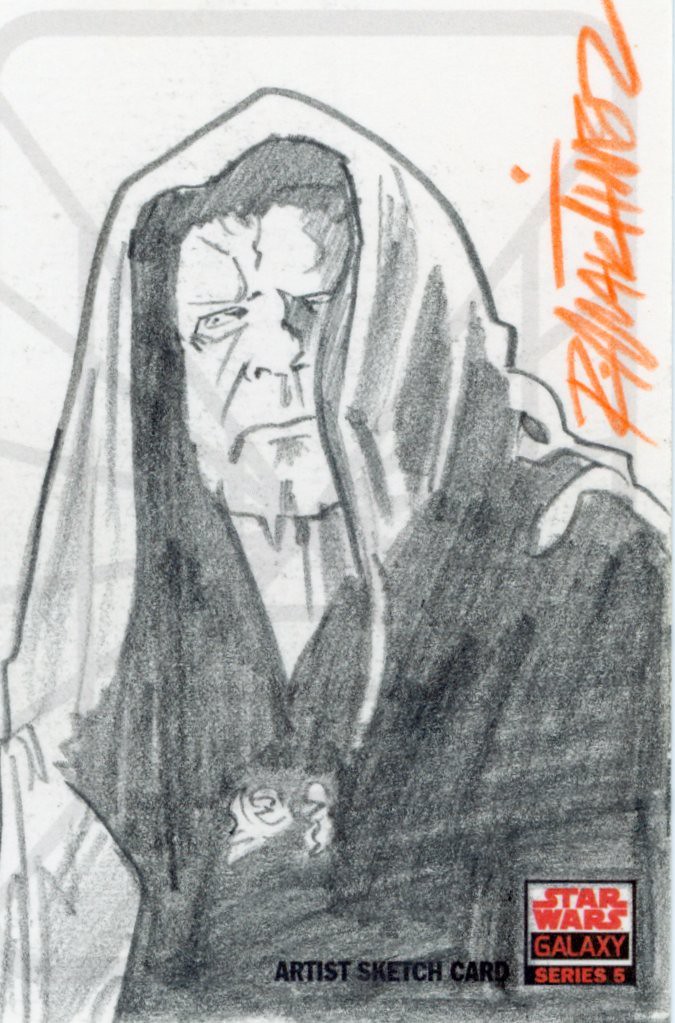This detailed sketch illustrates Emperor Palpatine, a notorious villain from the Star Wars saga. The character is rendered entirely in pencil, with extensive shading that captures his menacing presence. Palpatine is depicted wearing his signature long, dark cloak. The background oscillates between white and black, intensifying the contrast of the figure. At the top of the sketch, the artist's signature, which appears to be R. Martinez, is subtly incorporated. Below the drawing, a line of black text reads "Artist Sketch Card," with "Star Wars Galaxy Series 5" in red. An additional element in the top right corner includes some orange text, though its content is unclear. Despite the critique of its amateurish style and unrealistic details, the sketch encapsulates the dark essence of Emperor Palpatine.